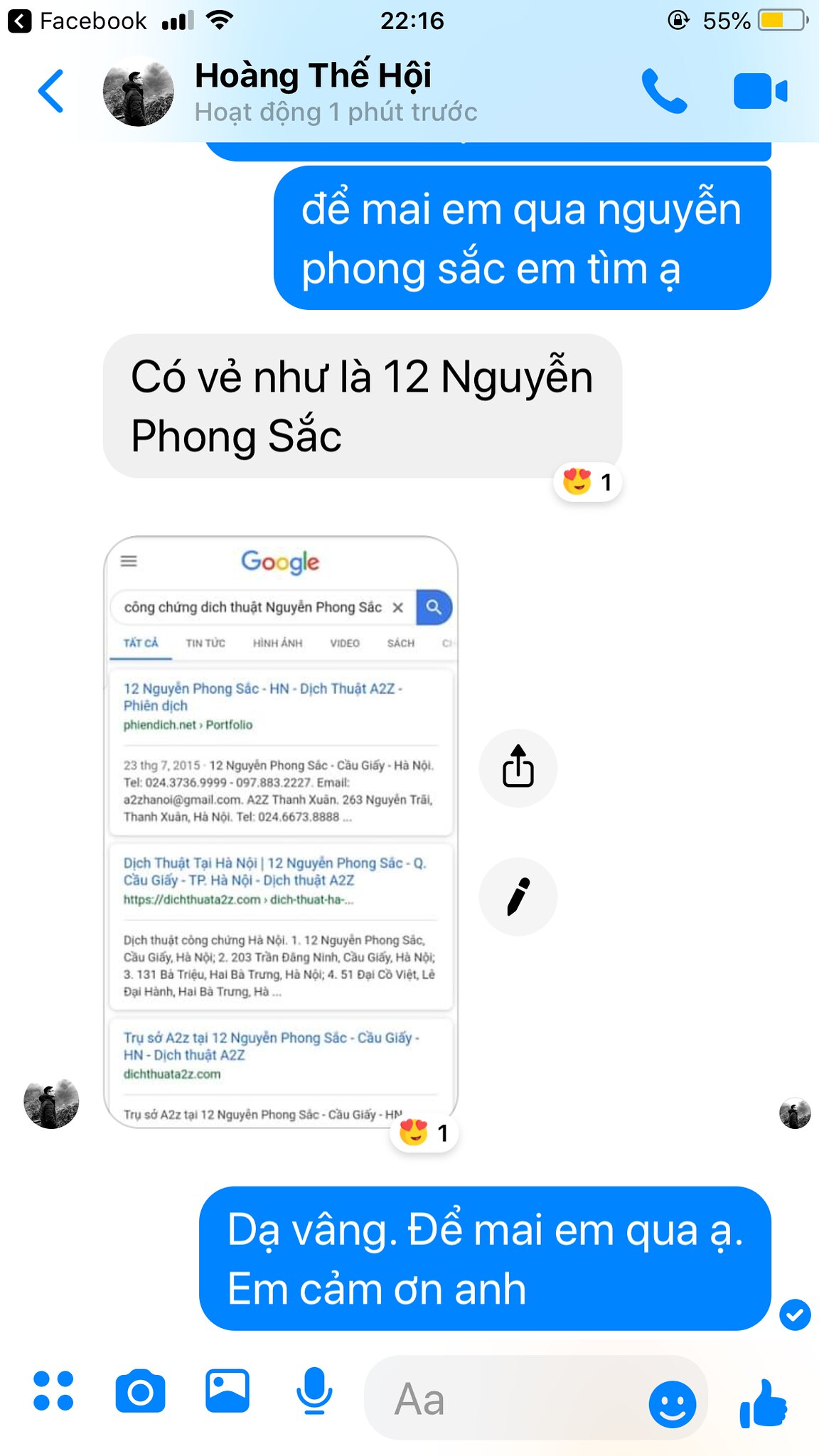This image is a detailed screengrab of a Facebook chat message log taken from a smartphone. At the very top left, it displays the Facebook logo adjacent to a circular profile picture and the name of the contact in a light blue band. To the right of the name are telephone and movie camera icons. Above this section, the top middle shows the time as 22:16, while the top right features a half-full yellow battery icon displaying 55%. Beneath this, the screen contains multiple text bubbles with white and black text written in a foreign language; the blue ones exhibit white text, and the gray ones display black text. Included in this sequence is a screenshot of a Google search result, with someone having reacted to it with a heart-eyed emoji. Below the text bubbles, a blue input bar with white letters appears, accompanied by various icons: a square, a camera, picture, microphone, smiley face, and thumbs up.